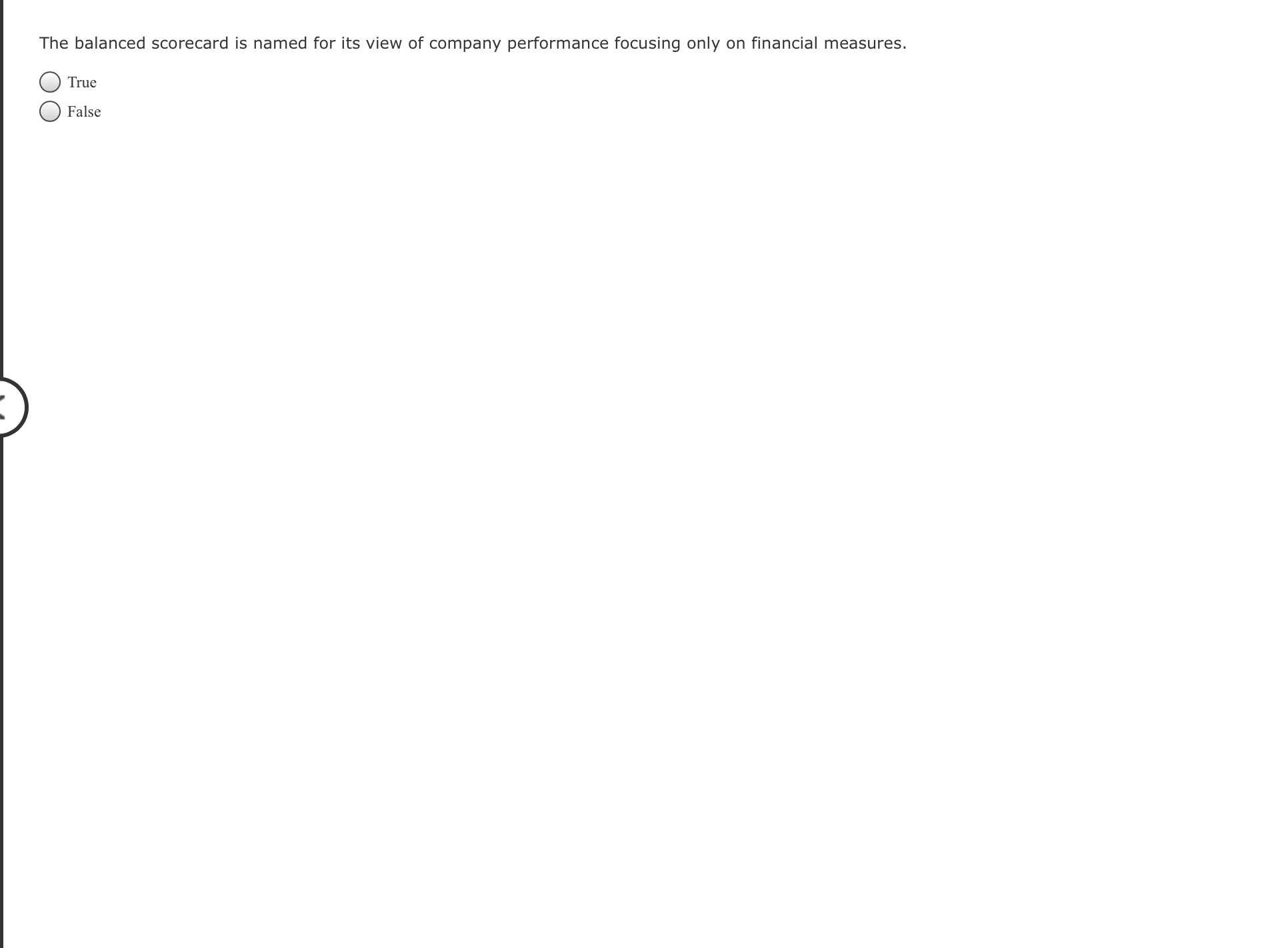This image depicts a true/false question displayed on a digital device. The question, presented in bold black letters on a white background, reads: "The Balanced Scorecard is named for its view of company performance focusing only on financial measures." Below the sentence, two gray circular buttons delineated with a thin black line are positioned. The button on the left is labeled "True," while the identical button on the right is labeled "False." The entire screen is predominantly white, except for a unique vertical line on the left side. This line extends a bit above the word "The" in the question, runs vertically downward, and has an intricate design including small curves and two dots resembling a face, before continuing as a dotted line toward the bottom.